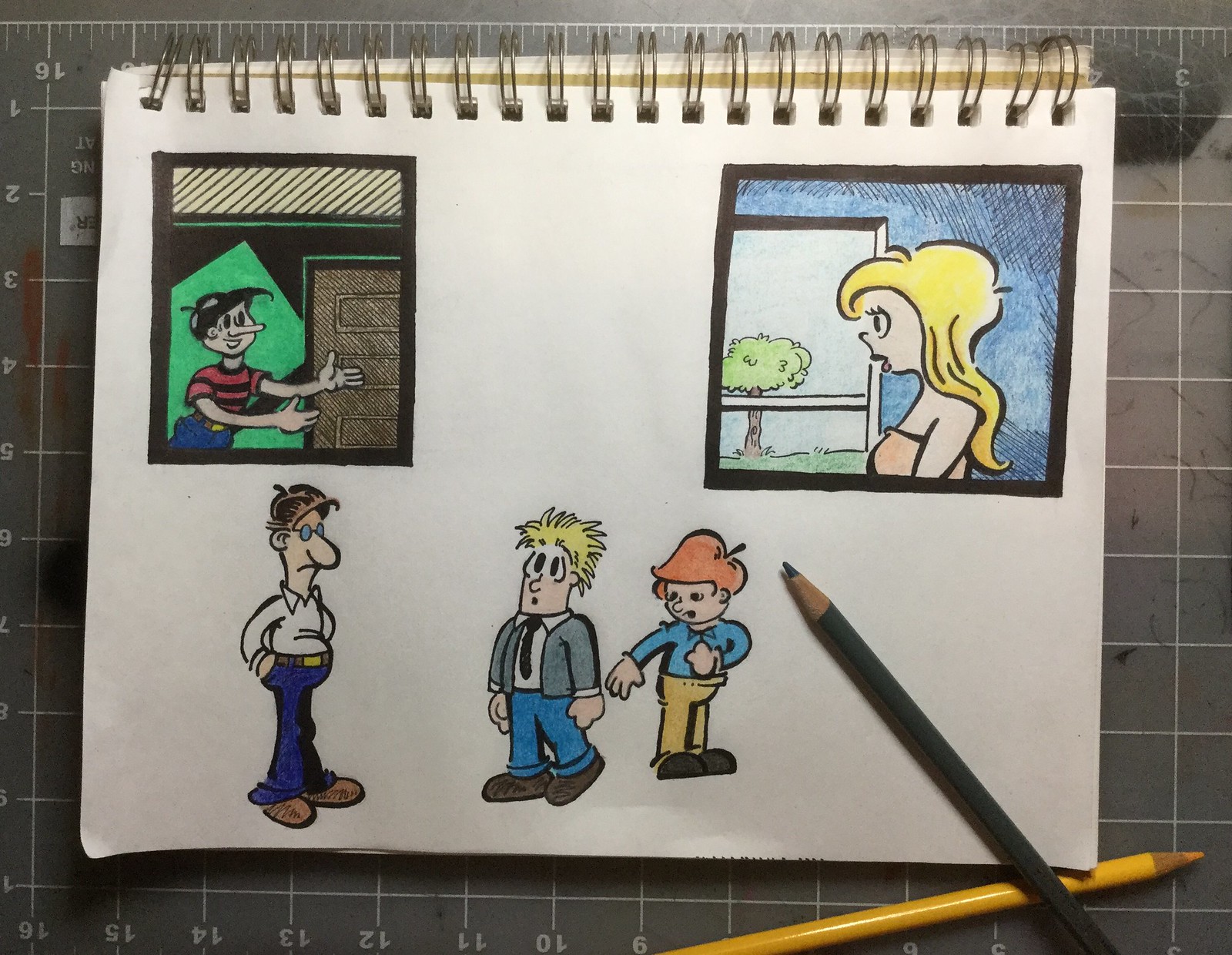The image depicts a first-person POV of a comic strip style drawing on a white sheet of paper, which is part of a sketchbook with a gold-colored binding. The sketchbook lies on a well-used craft cutting mat with grids and measuring rulers on its edges. The colorful drawing is situated in the middle of the mat, surrounded by a black or gray and yellow pencil crayon, partially resting on the paper and extending out of frame.

The sketch consists of two black-bordered cartoon boxes at the top and three more characters at the bottom. In the upper right box, a blonde-haired woman, wearing an orange halter top, gazes out of her window at a tree against a blue wall. The upper left box features a man resembling Jughead from the Archie comics, sporting a black and red striped shirt, black hair, and a long nose. He stands next to a brown door with his hands positioned in front of him.

Below these boxes, three more cartoon characters occupy the bottom half of the page. On the left, a man with messy brown hair, a pot belly, and round spectacles wears a white collared shirt and blue pants. Next to him, a man with spiky blonde hair, a white collared shirt, black tie, gray jacket, blue jeans, and brown shoes looks surprised with wide-open eyes. To his right stands a boy with orange hair, dressed in a blue shirt and yellow pants, and wearing black shoes. The drawing is vibrant and intricate, capturing the essence of classic Sunday newspaper comics.